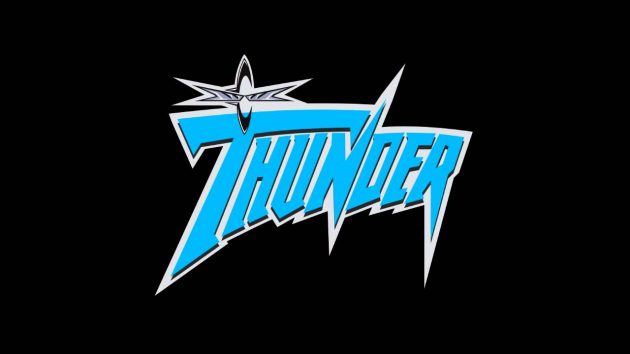The image features the word "THUNDER" in turquoise blue, capital letters with a slight slant to the right. The letter "T" extends its upper right part longer than usual, hovering over the subsequent letters. "N" contains pronounced spikes extending from its upper right and lower right parts, while "R" similarly extends downward with a sharp point at the lower right. The entire word is outlined or drop-shadowed in white, which makes it stand out against the pitch-black background. Above the letter "T," there is a logo in the shape of an unsettling face, encircled in black with a white face inside, adorned with grey glasses. The overall design is minimalist and dramatic, accentuating the contrast between the pale blue text and the dark backdrop.